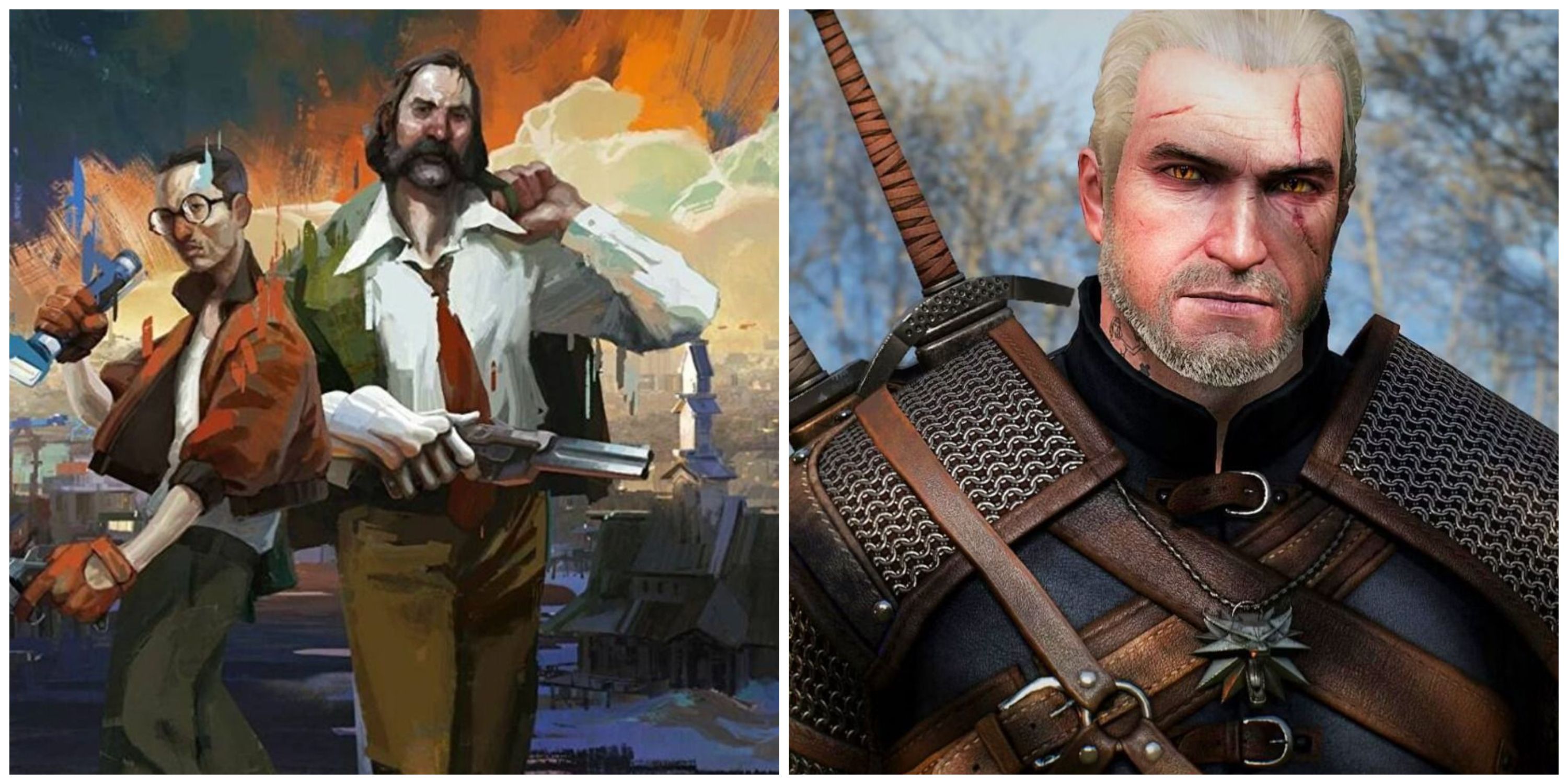This composite image features two side-by-side illustrations in a landscape orientation, appearing as stills from video games. The left illustration depicts two men standing before a city in ruins. The man on the left is shorter, sporting dark hair and round glasses with dark frames. He wears an orange bomber jacket over a white tank top, dark pants, and large orange gloves. He appears to be holding a blue-lit instrument. The taller man on his right has long brown hair styled in a bob and a thick, black mustache. He is dressed in a white button-up shirt, a red tie, dark pants, and a green jacket draped over his shoulders. His right hand, clad in a large silver glove, grips a large double-barrel gun.

The right illustration is a close-up of a character identified as Geralt from the video game The Witcher. He is depicted in medieval armor, complete with chainmail and leather-shoulder pads. Geralt has white hair pushed back, a short white beard, and piercing yellow eyes. His face bears distinct scars: one cutting through his eyebrow and extending down to his cheek, and another above his eyebrow. His armor features several leather straps, and a sword is visible strapped to his back.

The illustrations are colorful and detailed, capturing the essence of their respective video game worlds.